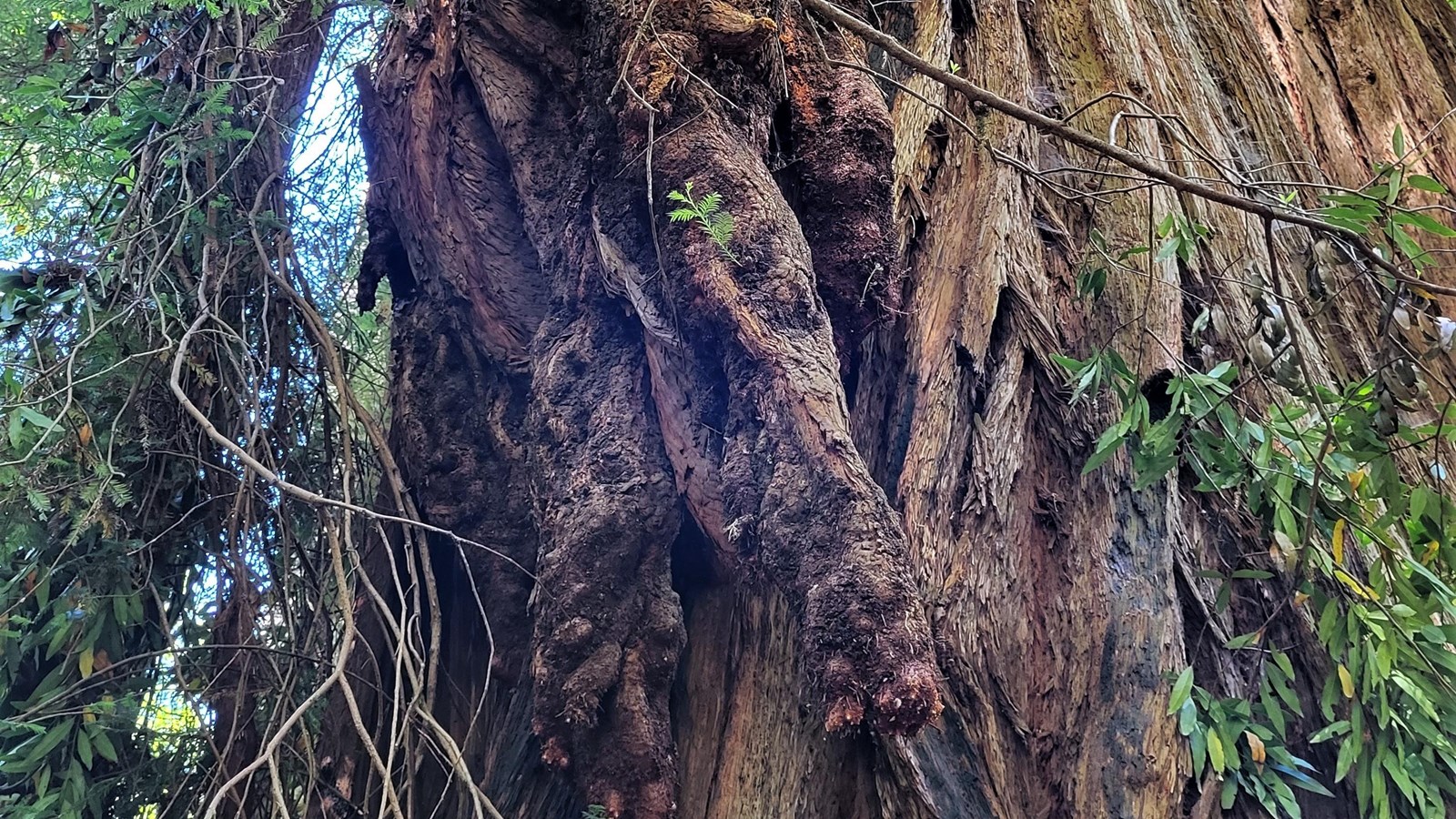The image depicts a large, thick tree trunk with a textured bark that has layers and twists, hinting at its impressive age and size. The trunk, colored in shades of light to dark brown, dominates the foreground and center of the shot. On the left-hand side, there are numerous green leaves and vines cascading downwards, adding a sense of lushness and natural growth. These leaves extend from the top left to the bottom left corner of the image. Overhead, a blue sky dotted with white clouds peeks through the foliage, indicating that the photo was taken during daytime. On the right side of the image, more vines or possibly branches with leaves are visible, twisting around themselves and adding to the intricate, layered appearance of the tree. The perspective of the photo is from the base of the tree looking upwards, capturing the grandeur and complexity of the trunk and overgrowth.